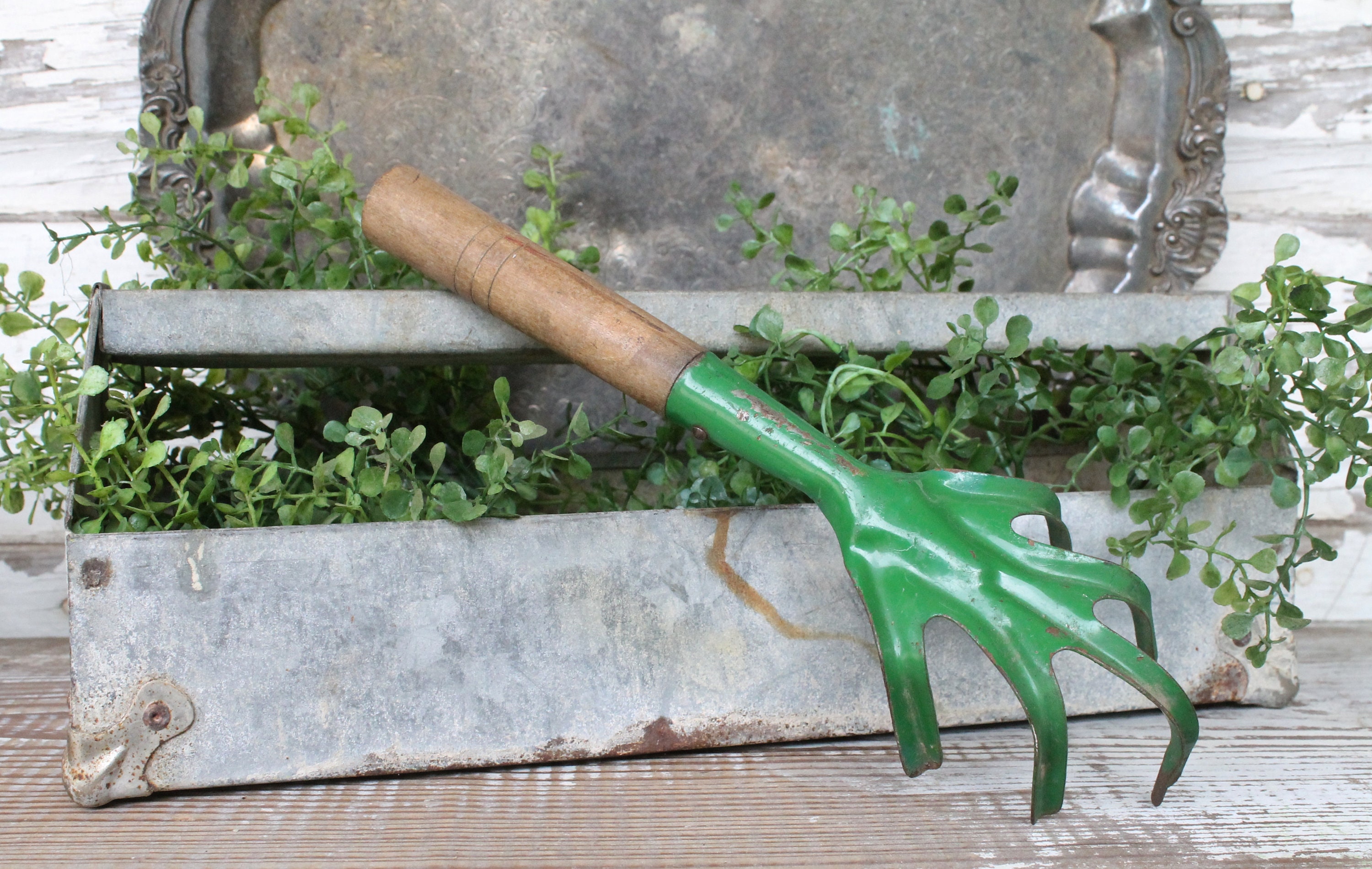The close-up horizontal image captures a rustic garden scene with intricate details. Central to the composition is a little hand rake used for planting, featuring a brown wooden handle and green metal prongs resembling fingers. This tool leans against an old, rusted toolbox-like container, which is horizontally rectangular and constructed of unpainted, light gray metal with brown spots of rust. The toolbox is filled with dense, thin branches adorned with tiny green leaves.

Behind the toolbox stands an oblong, tarnished silver platter, decorated with ornate crown molding trim and intricate engravings, reminiscent of early 1900s serving trays. The entire arrangement is set against a background of a wooden floor, which appears to have traces of white paint blended into the brown wood, adding to the weathered, vintage aesthetic. Overall, the scene conveys an old-world charm and a sense of history through its aged and well-used gardening tools and containers.